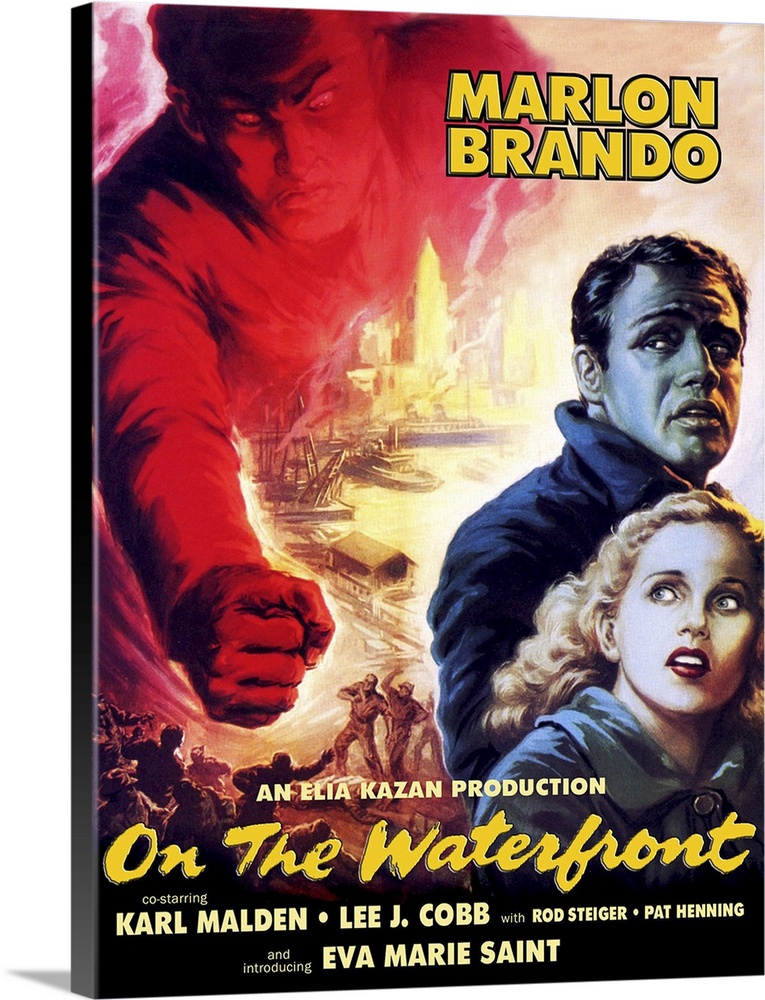The image is a movie poster for the film "On the Waterfront," presented on a wrapped canvas, lending it a vintage and textured appearance. The poster prominently features Marlon Brando's name in large yellow font at the top right, denoting him as the main star. It also credits the film as an Elia Kazan production, co-starring Karl Malden, Lee J. Cobb, Rod Steiger, and Pat Henning, with Eva Marie Saint making her debut.

The artwork depicts a dramatic scene set against the backdrop of a waterfront. Brando and a woman, likely Eva Marie Saint, appear on the right side of the image, both looking terrified as if something menacing is approaching. Above them, a large, sinister figure rendered in red with a hazy and smoky appearance looms ominously, representing the film's antagonist. The lower left section of the canvas shows a chaotic scene with men engaged in what looks like a mob or a battle, emphasizing the tension and conflict central to the story. The addition of indistinct fire or smoke elements adds to the overall sense of danger and urgency in the poster.